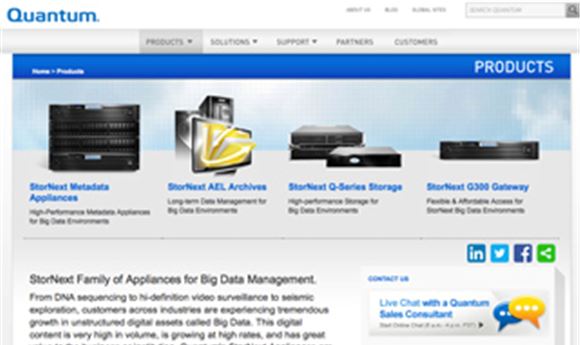Caption: 

The image features a predominantly blue-themed webpage from a company named "Quantum," with the title placed at the top left in bold blue letters. Adjacent to it on the right, there's a section titled "About Us," though the text following it is blurred and unreadable. A search box accompanied by a microscope icon is positioned below. Below the search box, a grey-highlighted menu bar displays the following categories: "Products," "Solution" with a down arrow, "Support" with a down arrow, "Partner and Customers." 

Further down, a blue background sharply contrasts with white text that labels various product categories:

- *StorNext Metadata Appliances"
- *StorNext AEL Archives*
- *Q5 Series Storage* 
- *G300 Gateway*

An additional section below these product listings provides a concise overview of the "StorNext" family of appliances, designed for big data management. It highlights their applications in diverse fields such as DNA sequencing, high-definition video surveillance, and realistic exploration. The description emphasizes that customers across various industries are witnessing significant growth in unstructured digital assets, commonly referred to as big data. This type of data is marked by its high volume and rapid growth rate, though the text cuts off abruptly.